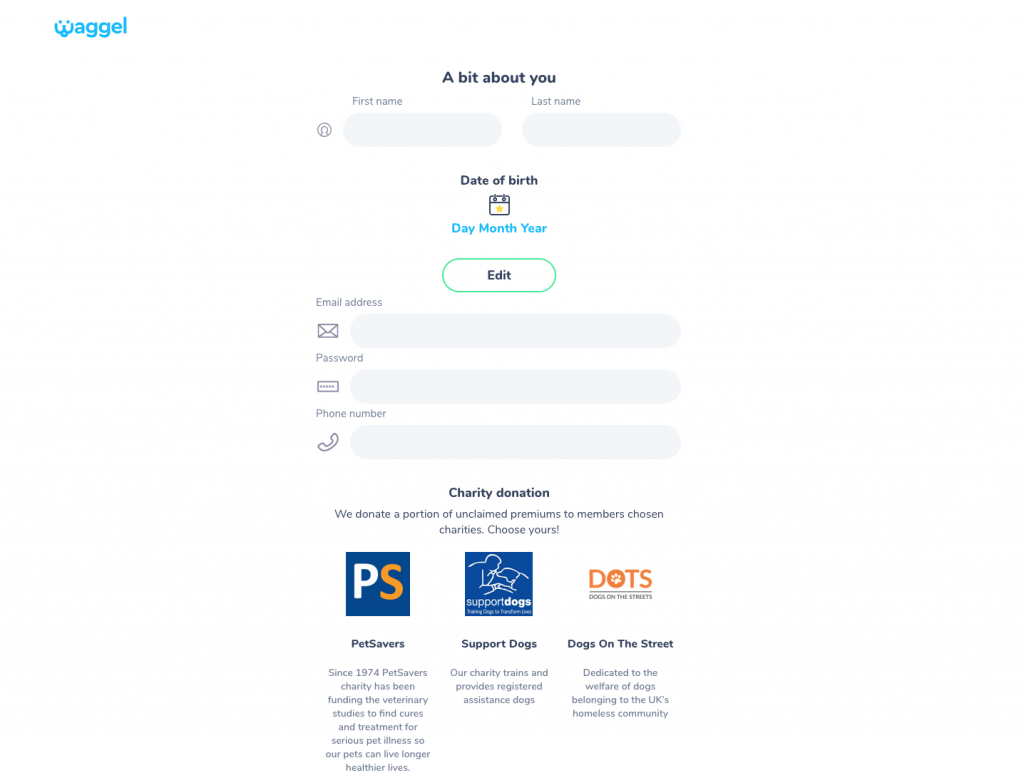The image is a screenshot of a webpage with a clean white background. In the upper left corner is the logo "Waggel," styled in blue lowercase letters. The 'W' is creatively designed to resemble a dog's face, complete with two dots above it representing eyes and a small half-circle suggesting a tongue, making for an ingenious logo.

Centrally displayed on the page is a narrow signup form with a light gray header that reads, "A bit about you." The form is segmented with several fields for user input. At the top, there are two adjacent rectangles designated for entering the first name and last name, followed by a field for the date of birth. Below these is a rounded-corner button labeled "Edit." Further down, three rectangles with soft, rounded corners are lined up, lightly shaded in gray, meant for the email address, password, and phone number.

Beneath these input fields is a section titled "Charity Donation," explaining that Waggel donates a portion of unclaimed premiums to charities chosen by its members. Users are prompted to "Choose yours" from three listed options:
1. **Pet Savers**: Represented by a blue square with a white 'P' and an orange 'S.'
2. **Support Dogs**: Identified by a blue square featuring a simple, stylized white line drawing of a man and a dog, accompanied by the text "support dogs."
3. **Dogs on the Street (D.O.T.S)**: Illustrated with a white square displaying the acronym D.O.T.S in orange, where the O contains a small dog paw image.

This detailed layout ensures clarity and ease of navigation for users signing up and selecting a charity of their choice.